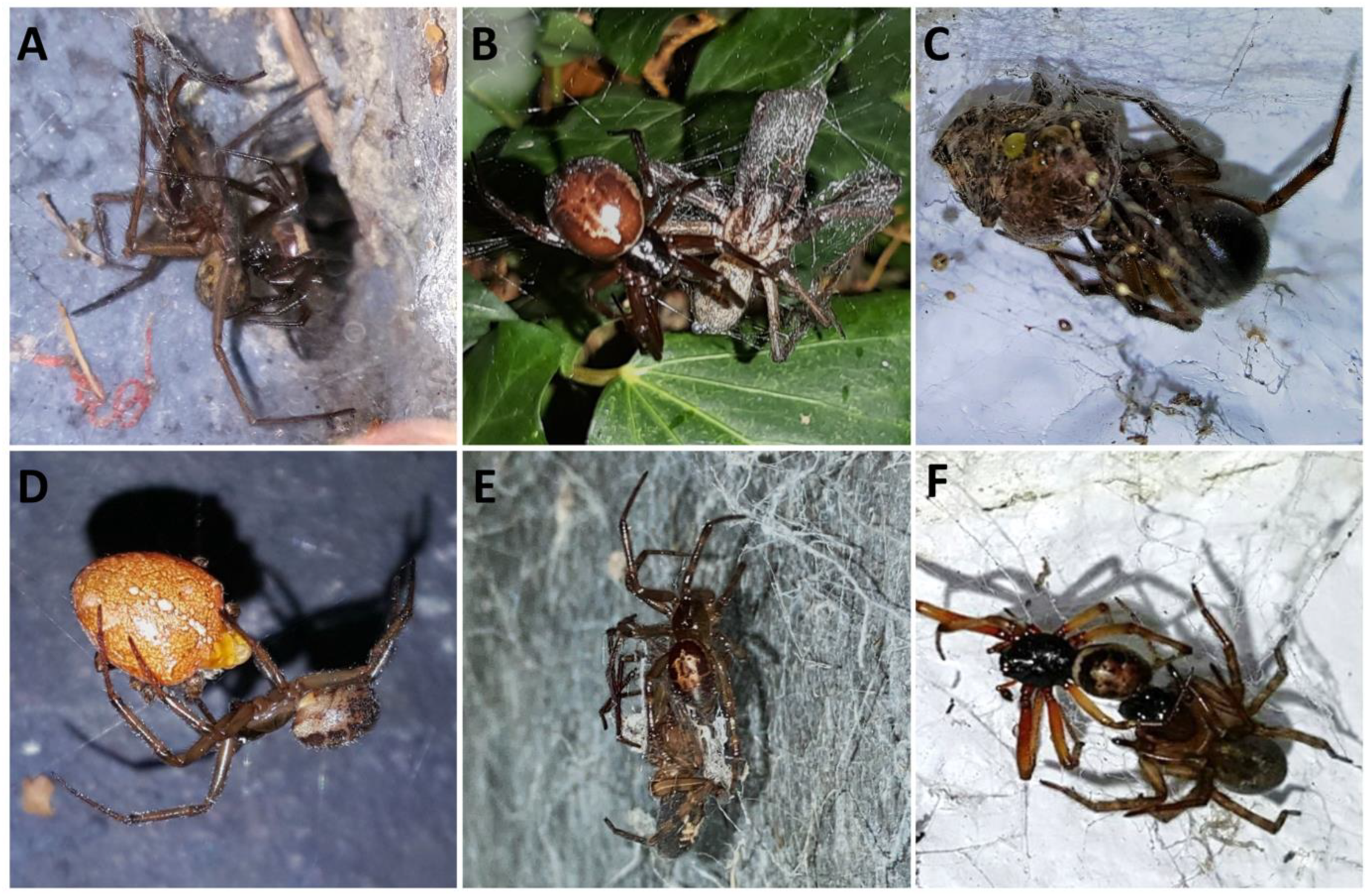This is a six-panel grid displaying various spiders, labeled A to F, from top left to bottom right. 

In panel A, a brown spider with long legs rests on a gray surface. Panel B features two spiders on green leaves; one has a brown abdomen, and another appears to be capturing its prey in a web. Panel C presents a black-and-brown spider on a gray background, seemingly feasting on an insect. 

Panel D shows a brown spider interacting with an orange object. Panel E, against another gray backdrop, displays a brown spider with darker legs, seemingly devouring another spider. Finally, panel F depicts two brown spiders with caramel-colored legs and black abdomens, possibly engaged in a combative stance with their legs interlocked.